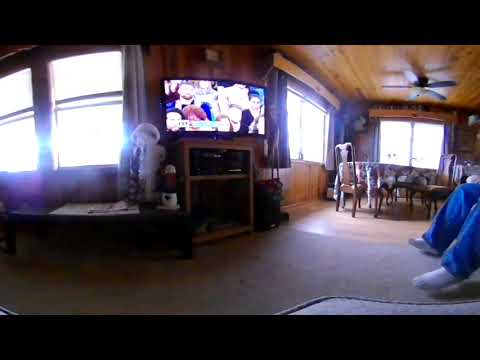The image features a brightly lit flat-screen television mounted on a wooden cabinet, positioned close to a wooden-colored wall. The television, bordered by a black frame, displays a vivid scene featuring a group of people, possibly an audience watching a talk show. The living room boasts a wooden ceiling adorned with a ceiling fan on the right side. To the left, three large windows allow natural light to flood in, with one particular window divided by a central frame into two panes. In the bottom right corner, a pair of legs clad in blue jeans and white socks extends towards the TV, resting on a light gray carpet. Further to the back on the right side of the image, a dining table covered with a floral-patterned tablecloth is surrounded by several chairs, placed against the windows. The overall setting, likely a living room inside a house, exudes a warm, daytime ambiance with a mix of wooden and carpeted flooring.